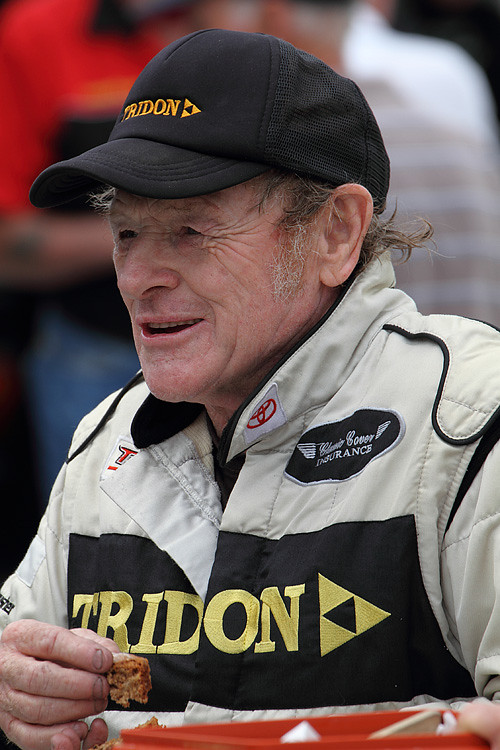This image captures a close-up shot of an older man facing slightly to the left. Highlighting the intricate details of his appearance, he wears a black baseball cap with orange writing across the front. His short hair is a mix of gray and brown, with noticeable white sideburns peeking out from under his cap. His facial features are marked by wrinkles, adding character to his expression.

The man's attire includes a heavy white and black jacket. Prominently displayed on the chest area is a black rectangle with the word "Tridon" written in yellow, alongside a triangle symbol. Above this emblem on the left side of his chest, there's a black patch with some writing on it. Additionally, a small Toyota symbol is visible on the collar of the jacket.

He is holding what looks like a piece of food in his left hand, with a possible tray positioned to the right of his hand within the frame. Although the photograph cuts off below his hand, the scene suggests he might be enjoying a meal, perhaps at a sporting event. The blurred figures of two people can be seen in the distant background, positioned at the upper left and right corners of the photograph, adding depth to the image's environment.